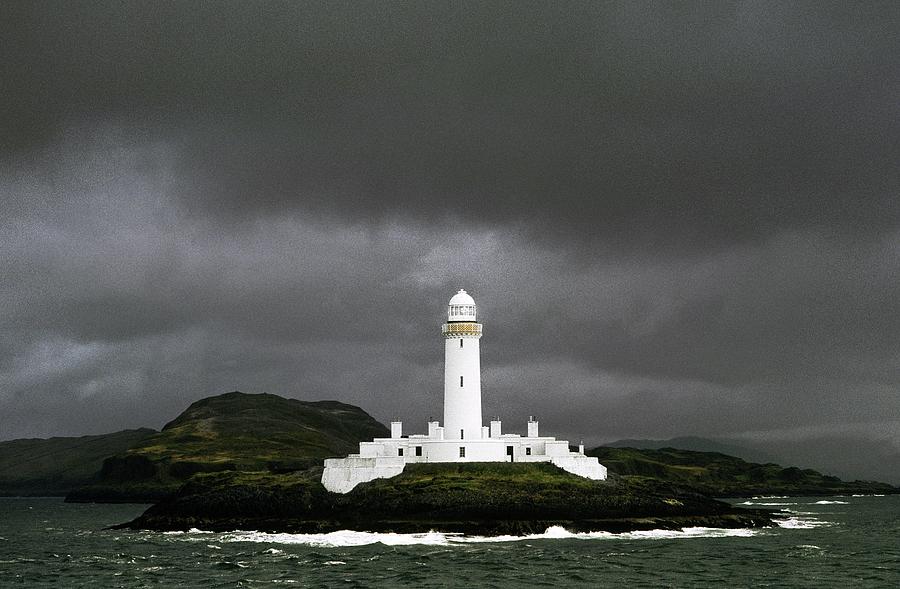In this atmospheric photograph, taken from across a dark, stormy sea, a large, vivid white lighthouse stands prominently on an island surrounded by rolling green hills. The sky is filled with dark, ominous clouds that suggest rain is imminent or has just passed, casting a dramatic backdrop that contrasts sharply with the lighthouse. The water below, dark blue and turbulent, crashes fiercely against the grassy slopes at the base of the lighthouse, creating striking white splashes. The lighthouse itself is a substantial structure, featuring attached white buildings that extend to its left and right, and a platform with steps leading down. While the lighthouse’s windows hint that one could enter, there are no lights currently shining from it. This highly detailed and zoomed-in image captures the stark contrast between the bright lighthouse and the brooding natural elements surrounding it, lending an almost surreal quality to the scene.